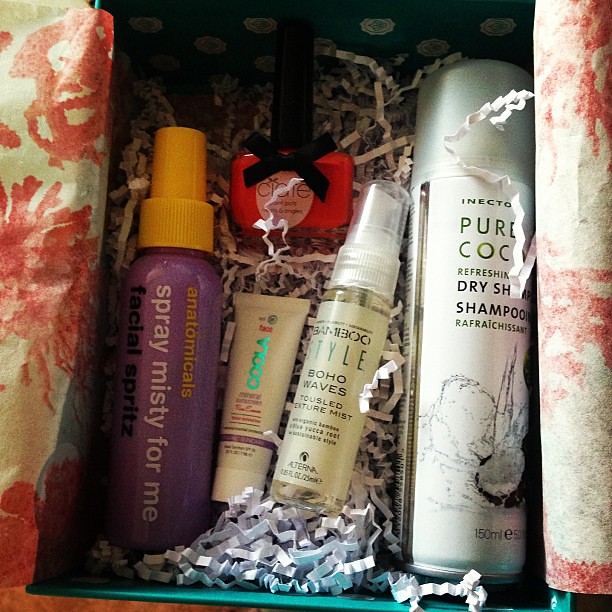The image displays an open gift box filled with self-care and beauty products, nestled in a bed of crinkled white paper strips with abstract red designs. The predominantly green gift box contains several items: a purple spray bottle with a yellow cap labeled "anatomicals spray misty for me facial spritz," a red nail polish with a black cap and ribbon marked with "C.R.A," a white bottle labeled "Kula" in blue, a white spray bottle inscribed with "bamboo style boho waves tousled texture mist," and a large white aerosol can with splashes of water and coconuts that reads "Insecto pure cocoa refreshing dry shampoo." The assortment suggests a thoughtful selection of hair and facial care items, perfect for a pampering session.